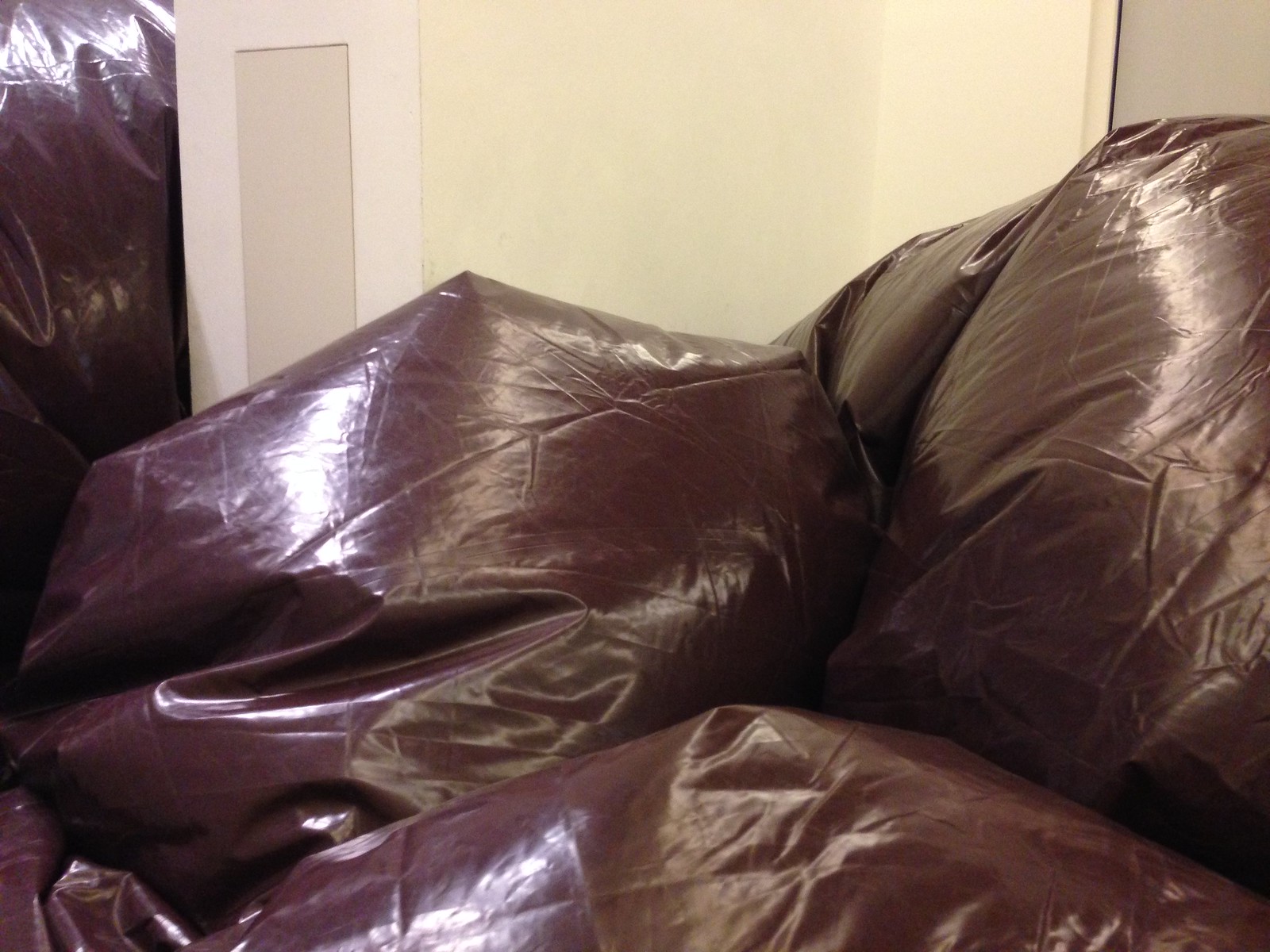This detailed photograph presents an indoor setting, possibly a storage space or cupboard, with white and light chocolate-colored walls. The focal point is an ambiguous pile of dark, shiny, burgundy-colored items, possibly thick plastic, positioned in the center of the image. At first glance, these items could be mistaken for a distressed leather sofa with worn elements resembling baggy pillows, but closer inspection suggests they are more likely garbage bags or possibly bean bags due to their pronounced shiny texture and how they glisten under the light. At least four of these bags are clearly stacked atop one another, with an additional one partially visible in the upper left corner. In the middle of the frame, a white wall surface can be seen, alongside a gray square in the upper right-hand corner, likely a part of the wall. The obscured view adds to the ambiguity, suggesting the contents could be anything from duvets, clothes, or towels, typically found in a hotel or storage scenario, to miscellaneous items awaiting transport.